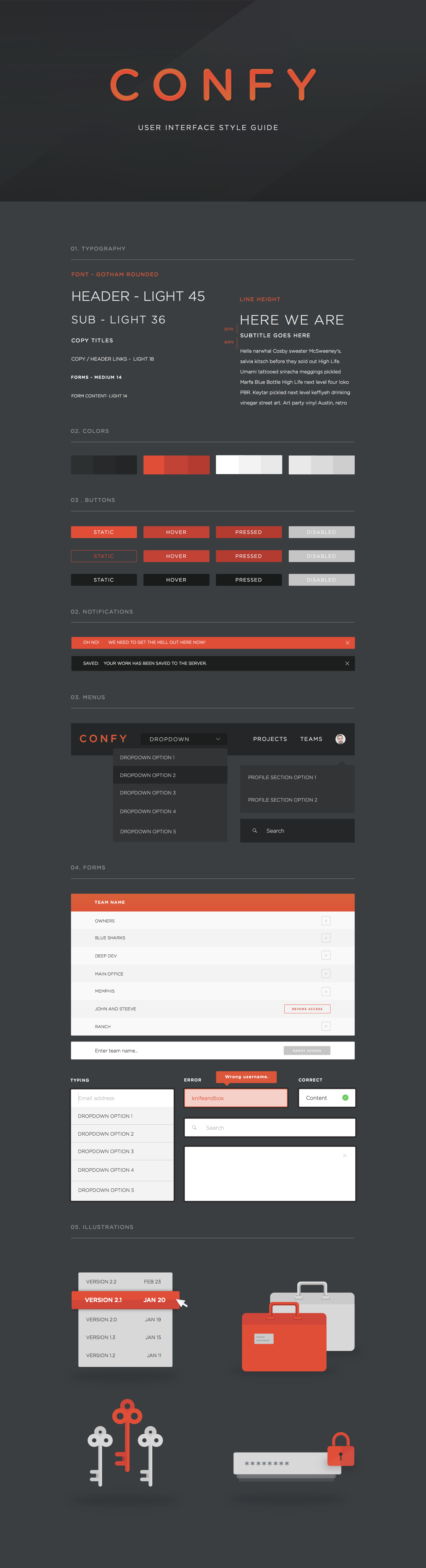This image is a detailed screenshot of a large webpage. The webpage prominently features the title "CONFY," spelled out in bold, capitalized letters in a vivid red font at the very top. Below this prominent heading lies a small, illegible description of the website's content. Scattered across the page are various buttons in three different colors: red, white, and black.

Towards the lower section of the page, there are multiple white input tables, suggesting areas where users can enter specific information, though the text and input fields are too small to read clearly. The bottom-left corner of the screenshot displays an image of three keys positioned side by side. The central key is a dark orange, almost red, while the two keys flanking it are white.

The entire webpage is set against a dark gray background, adding a stark contrast to the elements in the foreground.